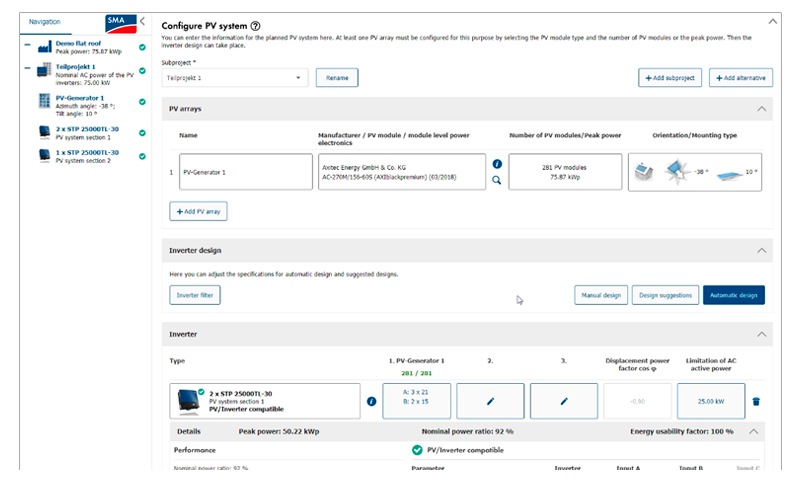A plain white desktop web page with a simple design. On the left side, there's a vertical menu entitled "Navigation," featuring a red and blue, credit card-shaped logo for the company SMA. The menu includes various options and small images of different products, each annotated with green tick marks beside them. Due to the blur in the image, the text within the menu is difficult to read.

The main content area, occupying about four-fifths of the page, is dominated by configuration options for photovoltaic (PV) systems. The page title, "Configure PV Systems," indicates the primary purpose of the site—allowing users to customize and configure solar panel systems. Sections listed include "PV arrays," "inverter design," "inverter," and "details," each with options for detailed customization. The overall layout is functional but lacks aesthetic appeal, characterized by small text and minimal, small images.